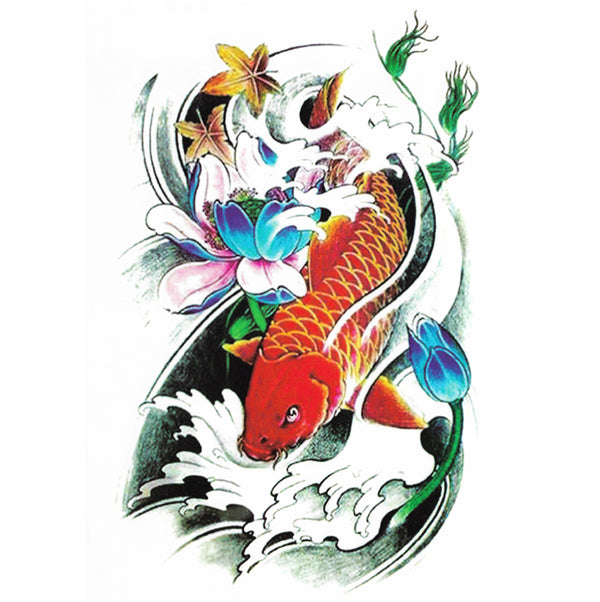This intricate painting features a vibrant red koi fish adorned with yellow scales and yellow fins, swimming with intense focus suggested by its downward-pointing whiskers and concentrated eyes. The fish is enveloped in dynamic white waves that create a sense of motion and energy. Surrounding the koi are various floral elements, including prominent blue flowers with purple tips and white interiors, some of which appear layered above and below the fish, enhancing the complexity of the composition. Additionally, there is a green stem with a blue bud at the lower right, and five-pointed golden leaves scattered throughout, mingling with green seaweed in the upper right corner. The background is an off-white color, devoid of clear borders, invoking the style of a sophisticated and abstract tattoo design. Through its multiple layers and interwoven elements, the artwork achieves a harmonious and meticulously planned arrangement.